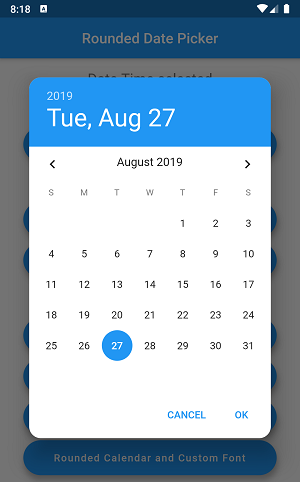This image is a screenshot taken at 8:18 of a calendar page displayed on a phone, captured from another phone. On the screen, an application resembling WordPad is visible, with its interface indicating full Wi-Fi signal, full cellular bars, and a fully charged battery.

Dominating the screen is a date-picker interface with a blue header bar featuring white text. The upper section of the interface displays the date "Tuesday, August 27, 2019" in a blue bar. Below this, the calendar shows the month of August 2019 against a predominantly white background. The current date, the 27th, is highlighted with a blue circle.

Towards the bottom of the interface, there are two buttons: "Cancel" and "OK," both imbued with a blue background and white lettering, adhering to the rounded design theme of the date-picker. The remainder of the screen, occupied by the calendar menu, conceals additional application buttons, making them indistinguishable. 

The screenshot's context implies that the user is attempting to set an event on Tuesday, August 27, 2019.